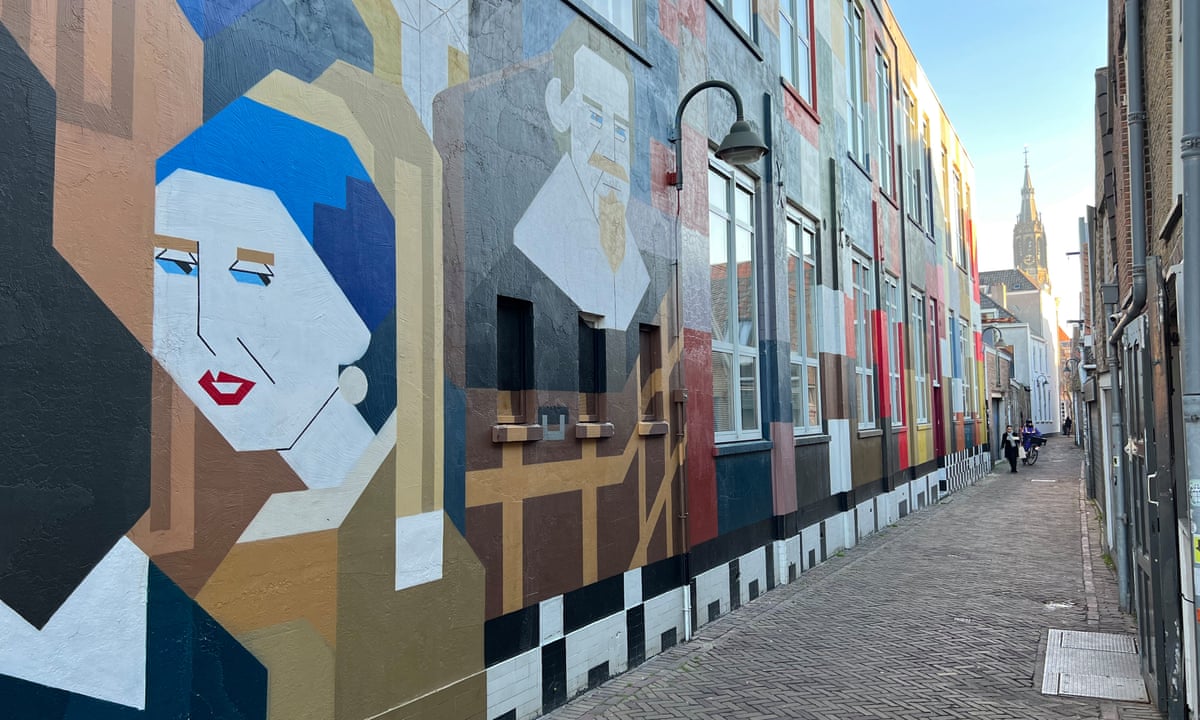The photograph captures a vibrant, brick or cobblestone-paved narrow walkway flanked by two-story buildings with flat roofs, likely in a European city, possibly Holland. The left side of the walkway is adorned with a series of colorful murals extending the entire length of the buildings. Prominently featured in the foreground is a modern, cubist interpretation of Vermeer’s “Girl with a Pearl Earring,” showcasing her blue eyes, red lips, blue hair, and iconic pearl earring. Behind her, there is a mural of a man with a goatee and beard, possibly resembling Vermeer himself or William Shakespeare.

In the background, a church spire is visible at the vanishing point on the right side, underneath a blue and white sky, adding a hint of historical architecture to the urban scene. Street lamps attached to the side of the buildings provide illumination, although this appears to be the less frequented back entrance of the buildings, given the absence of doorways.

A few human figures are seen walking up the clean, well-maintained street, adding a touch of life and movement to the scene.